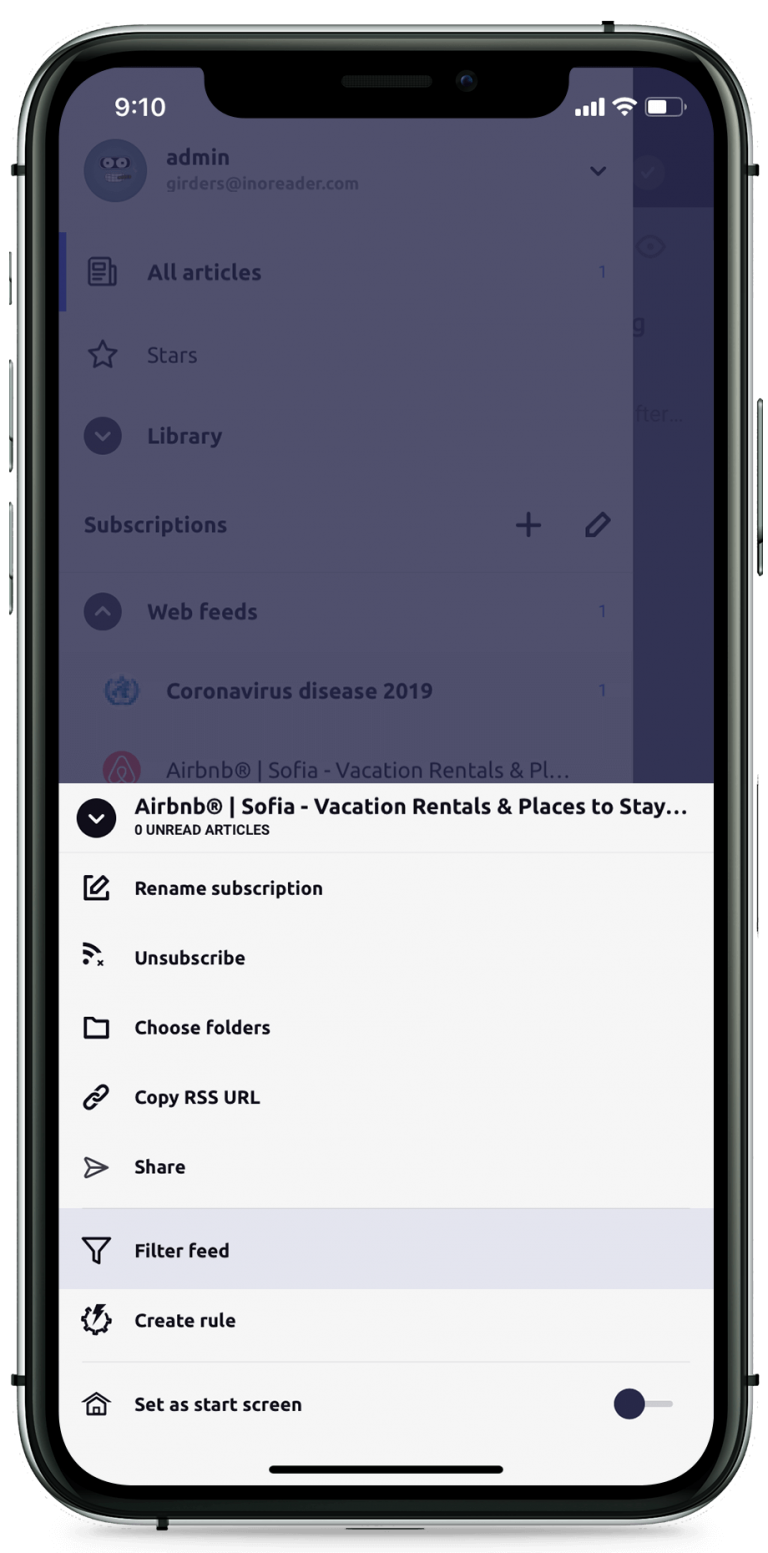The image displays a gray background with the status bar at the top showing a time of 9:10, four signal bars, a Wi-Fi signal, and a half-full battery icon. Below the status bar, there are tabs labeled Admin, All Articles, Stars, Library, Subscription, Web Feeds, Coronavirus Disease 2019, Airbnb, Sophia, and Vacation Rentals.

Beneath these tabs, within a white box, the text Airbnb, Sophia, Vacation Rentals, and Places to Stay is displayed. Further down the image, each line consists of an icon on the left corresponding to a particular function on the right. The functions and their associated icons from top to bottom are as follows:

1. "Rename Subscription" with an icon of a piece of paper and a pencil.
2. "Unsubscribe."
3. "Choose Folders" with a folder icon.
4. "Copy RSS URL" with a paperclip icon.
5. "Share" with a paper airplane icon.
6. "Filter Feed."
7. "Create Rule."
8. "Set As Start Screen" with a left-facing toggle switch icon.

The icons clearly represent the actions they accompany, providing a visual guide to the different functions available.